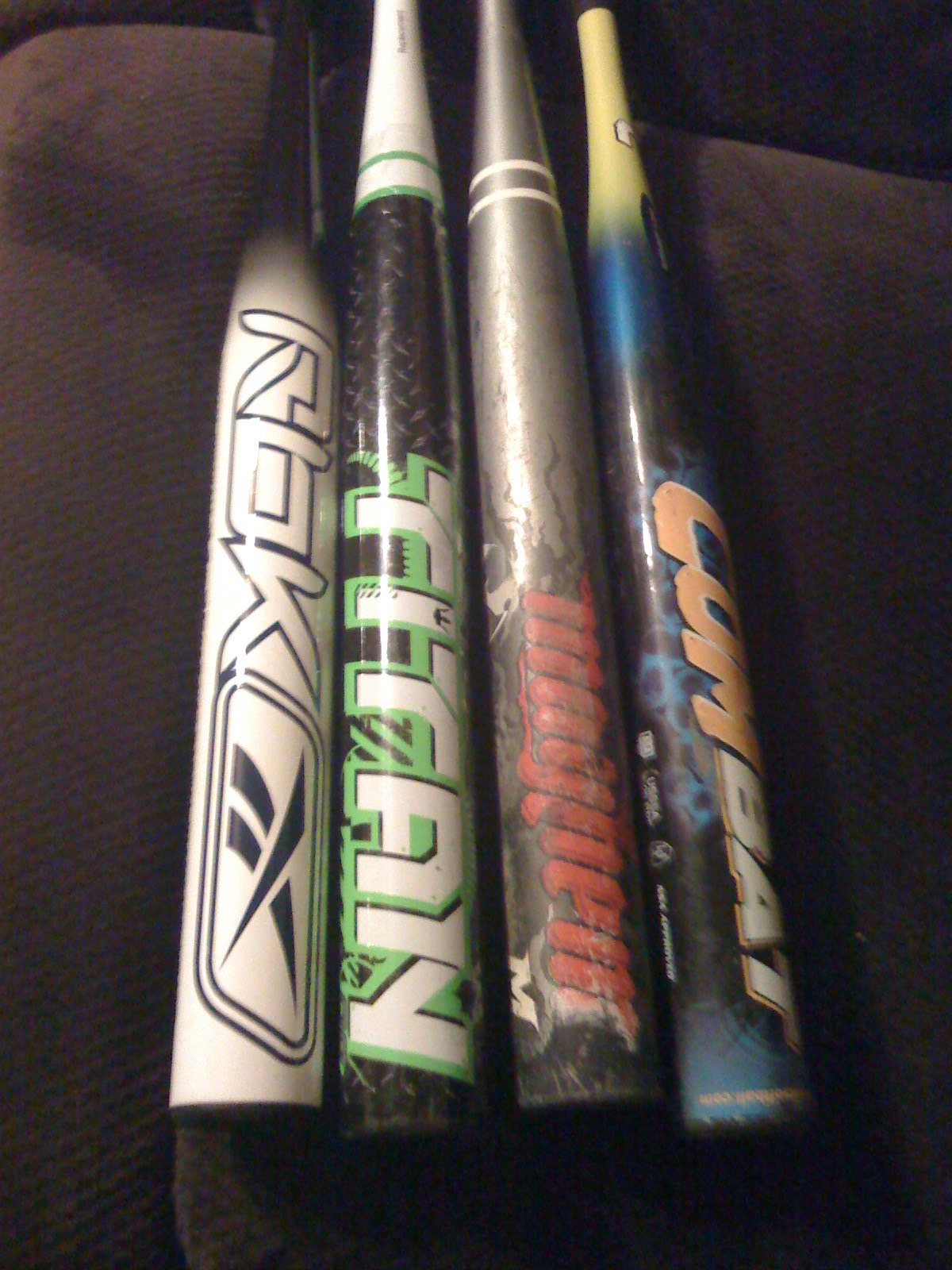The photograph depicts the lower portions of four baseball bats arranged side by side on a dark brown, slightly patterned upholstery, suggestive of a couch or chair. The bats are shown with their handles oriented upwards at the top center of the frame, and the ends that strike the ball facing downwards. 

From left to right:
1. The first bat is predominantly white with a prominent black and white logo displaying the letters "RBK" and a possible Reebok symbol.
2. The second bat features a black base with green and white lettering spelling "TITAN," framed with an iron grate-like pattern.
3. The third bat is a silver-gray with white circular rings and has red lettering, possibly spelling "MAGNEM."
4. The fourth bat showcases a striking gradient from yellow towards the handle down to black and blue, embellished with a combination of blue lightning designs and orange-turned-white "COMBAT" lettering.

All four bats appear to be well-used, exhibiting a variety of color schemes and logo designs.